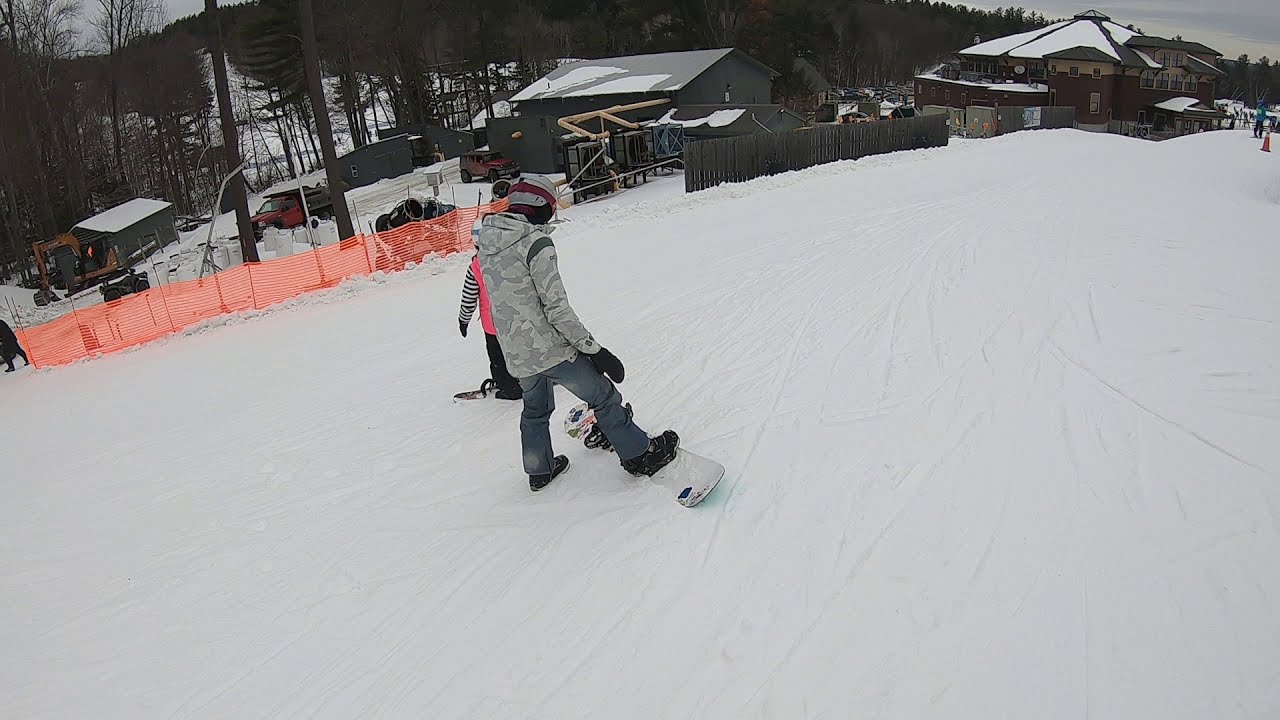In this vibrant landscape-oriented photograph, captured as a GoPro video freeze frame, two snowboarders are preparing to descend a snow-covered slope. Both individuals face away from the camera, with the nearest wearing dark grey snow pants and a light grey camo-style winter jacket, accented by black gloves. Slightly behind and to the side, a smaller, possibly younger, snowboarder dons a pinkish jacket with black and white sleeves. The crisp, bright white snow blankets the ground around them, contrasted by the vivid orange plastic fencing and traditional wooden fencing lining the right side of the slope. Beyond the fences, the land slopes downward, revealing a couple of grey buildings with red trucks parked outside and, in the upper right corner, a large ski lodge-style building. The scene, bathed in realism, evokes the structured thrill of a ski resort, dotted with safety cones and hinting at a familial day of snowboarding amidst snow-laden trees and rooftops.